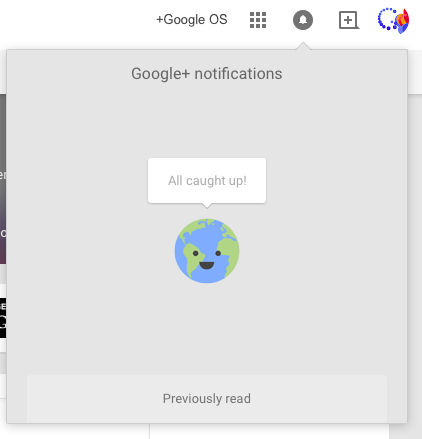The image depicts a Google Plus notification screen on a mobile device. In the top-right corner, there's a cluster of icons: a message bell logo, a nine-square tic-tac-toe styled grid, a square with a plus sign, and an intricate logo resembling the letter 'B' with red and orange hues, flanked by blue elements and circular blue dots. This iconography overlays part of the screen, which is partially obscured.

Dominating the foreground is the notification overlay— a gray semi-transparent field showing the Google Plus notifications interface. Central to this overlay is a simple graphic of planet Earth, adorned with a smiling face and a speech bubble stating, "All caught up!" in light gray text. Below this graphic, a peach-colored rectangular bar spans the bottom of the gray field, labeled "Previously read."

In the background, barely visible, are glimpses of the underlying screen, featuring some indistinct JPEGs, text snippets, and a vertical gray bar on the right. The rest of the visible screen is predominantly white. This detailed caption illustrates a moment of a user checking their notifications on Google Plus.